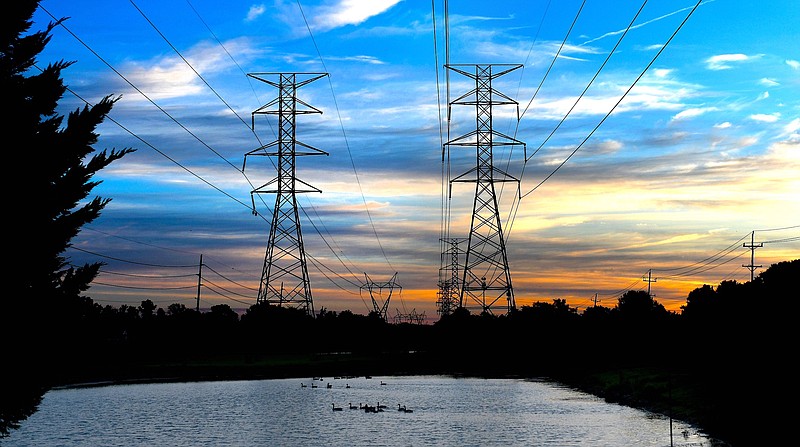This photograph captures a tranquil rural scene dominated by a steely blue-gray pond stretching from the left edge to partway across the right. The pond is inhabited by a family of ducks, their silhouettes trailing ripples in the water as they swim mostly leftward. Bordering the pond are silhouetted trees and plant life, including a tall pine tree extending to the top of the frame on the left, and lower vegetation clustered towards the bottom third of the picture. 

Dominating the center of the photograph are two prominent electrical towers with pyramidal bases adorned by a lattice of X-shaped supports. These towers hold four trapezoidal fixtures near their summits, three facing downward and one inverted, from which numerous power lines extend into the horizon. Additional smaller power lines run along both the left and right edges of the frame, with smaller and more distant towers visible as they recede.

Above this industrial landscape, the sky occupies about two-thirds of the frame, transitioning from a deep blue at the top to a warm orange near the horizon, interspersed with streaks of gray and yellow clouds. The time of day suggested by the sky's gradient hues indicates either early dawn or approaching dusk, adding a muted yet captivating spectrum of colors to the scene.